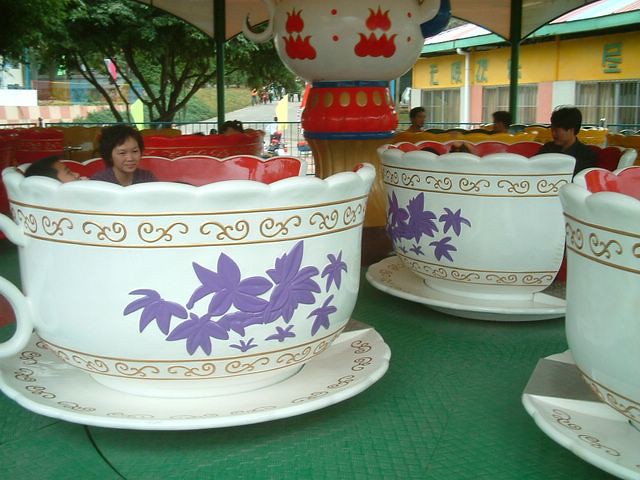The image depicts a vibrant teacup ride in an amusement park, filled with detailed ornamental features and lively activity. Each teacup is meticulously designed; they are white with gold trim accentuated by intricate leaves and vines, as well as clusters of delicate purple flowers, likely lilacs, adorning them. These lifelike teacups sit in matching white saucers on a green platform. The interiors of the teacups are strikingly bright red, adding to the ride's colorful appeal. The ride's center features a yellow tower with a red midsection embellished with gold dots, transitioning into a white top section adorned with red tulip designs, resembling the petals of a tulip. The ride canopy suggests it is likely located in China or Japan, supported by Japanese writing visible on several buildings in the background. The scene captures a large crowd of people walking along a pathway between the rides. Specific details include an Asian woman with short black hair in a blue shirt sitting next to a child inside a teacup, and an Asian man with short black hair and a dark-colored shirt in another teacup. The photograph showcases not only the intricate details of the ride but also the lively atmosphere of the amusement park, with patrons visible in teacups and background crowds.